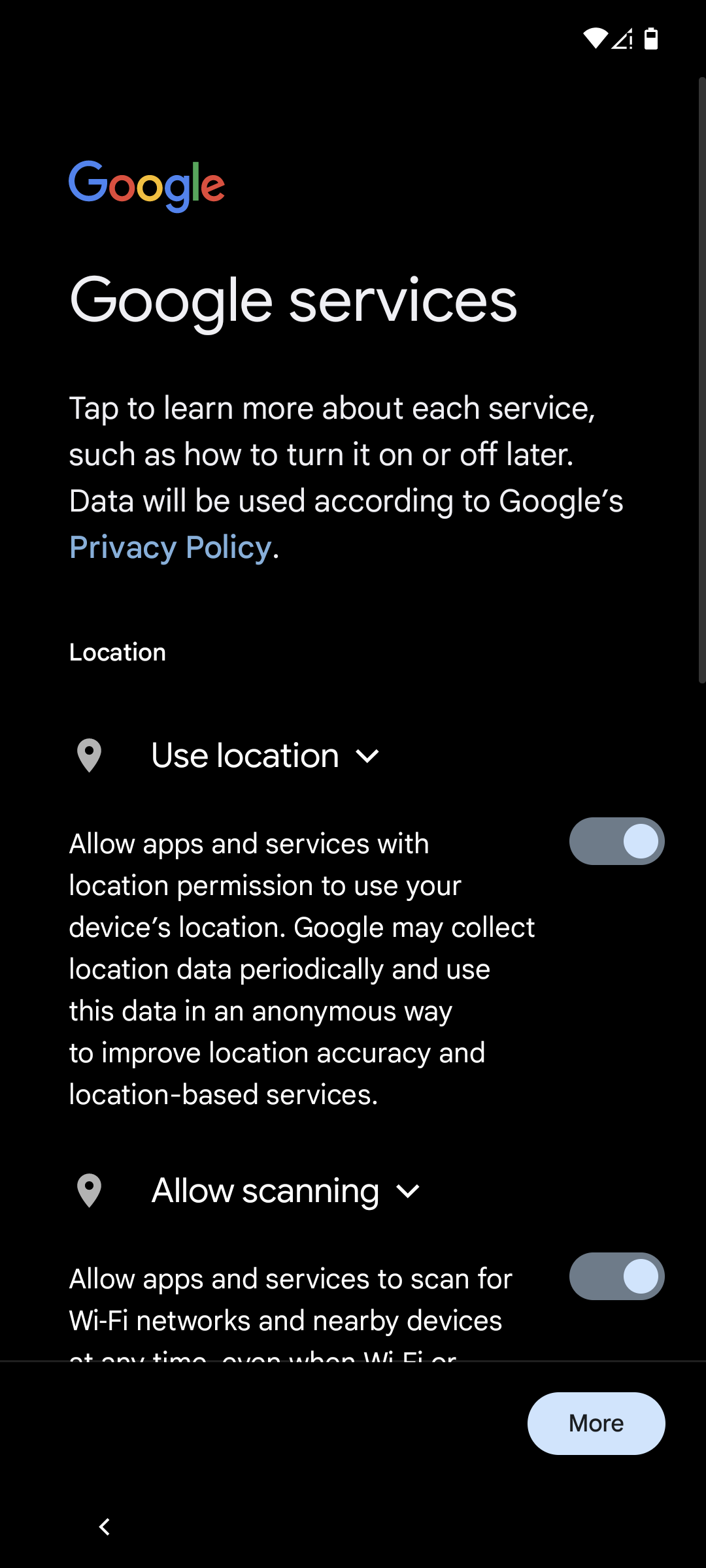The image appears to be a screenshot taken on a mobile device, either a phone or a tablet. At the top of the screen, there are indicators for Wi-Fi signal strength and battery life. Below that, the familiar "Google" logo is displayed in its characteristic multi-colored format: blue, red, yellow, and green. Just beneath the logo, in white text, the screen reads "Google Services". A brief instructional message follows, stating: "Tap to learn more about each service such as how to turn it on or off later. Data will be used according to Google's privacy policy."

Highlighted in blue text, the term "privacy policy" is likely a clickable link. Following this, the section on "Location" is detailed. It includes a toggle switch and states: "Use Location - Allow apps and services with location permission to use your device's location. Google may collect location data periodically and use this data in an anonymous way to improve location accuracy and location-based services."

In addition, there is another section labeled "Allow Scanning," which includes a description of what this feature does. Adjacent to each option, there are toggle bars that allow the user to turn these settings on or off.